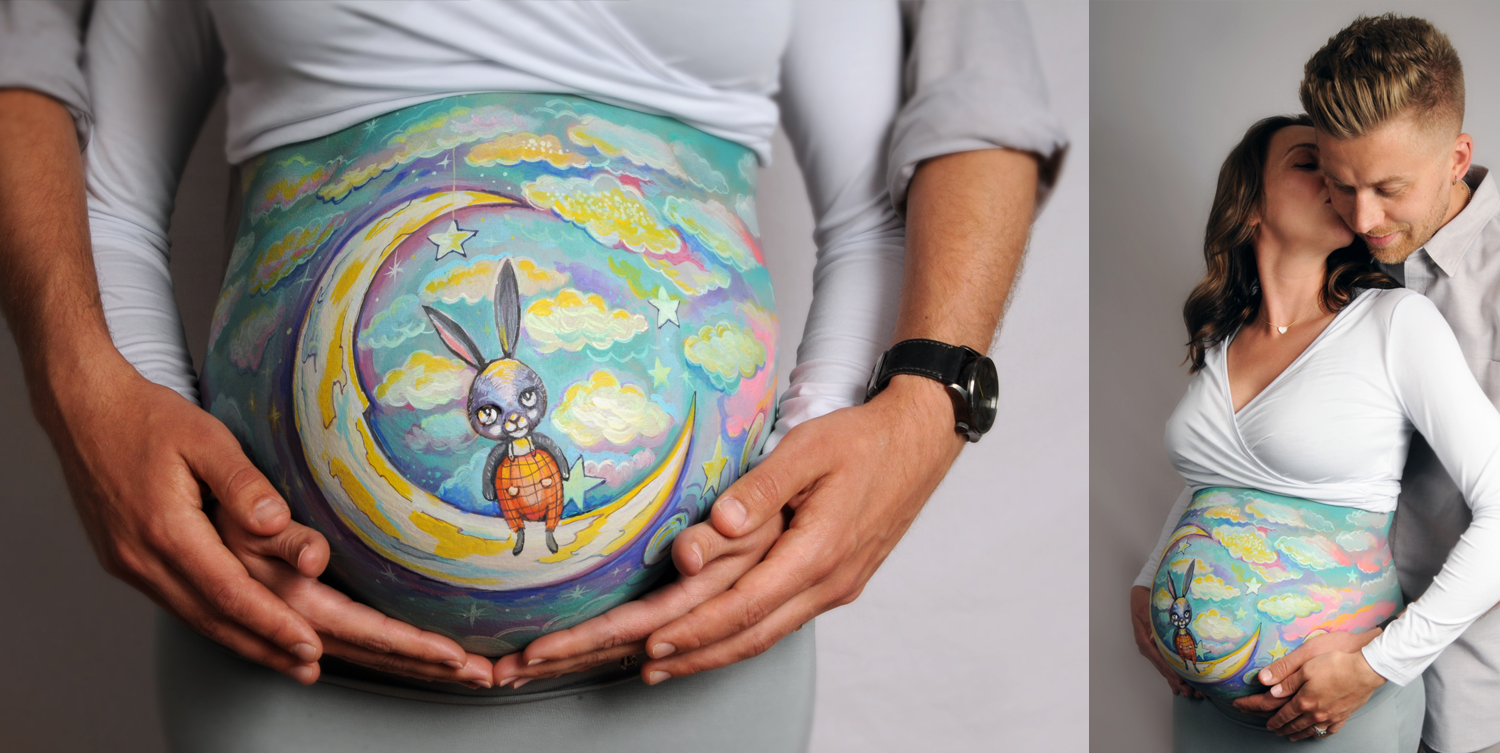This detailed composition features two side-by-side photographs of a loving couple, assumed to be the same individuals in both images. The larger photograph on the left, which occupies roughly 75% of the frame, showcases a pregnant woman revealing her artistically painted belly. Both participants are captured in a tender moment as she cradles her belly with her two hands above his. The intricate belly painting depicts a whimsical scene of a gray rabbit, adorned in orange overalls, perched on a crescent moon amidst a sky of blue and pink hues, dotted with white and yellow clouds, and a few stars. The woman is dressed in a white long-sleeve shirt, pulled up to reveal the artwork, while the man, identifiable by his rolled-up gray shirt sleeves and black watch, stands behind her with his hands gently placed on hers.

The smaller photograph on the right presents a waist-up view of the same couple sharing an intimate moment. The man, with his blonde hair styled upwards, smiles as the woman, with sandy blonde hair, sweetly kisses his right cheek. They are still dressed in the same attire, with the painted belly prominently featured. The consistent elements of their clothing and the beautifully painted belly, along with their tender interactions, suggest a strong bond and shared joy in anticipating their child.